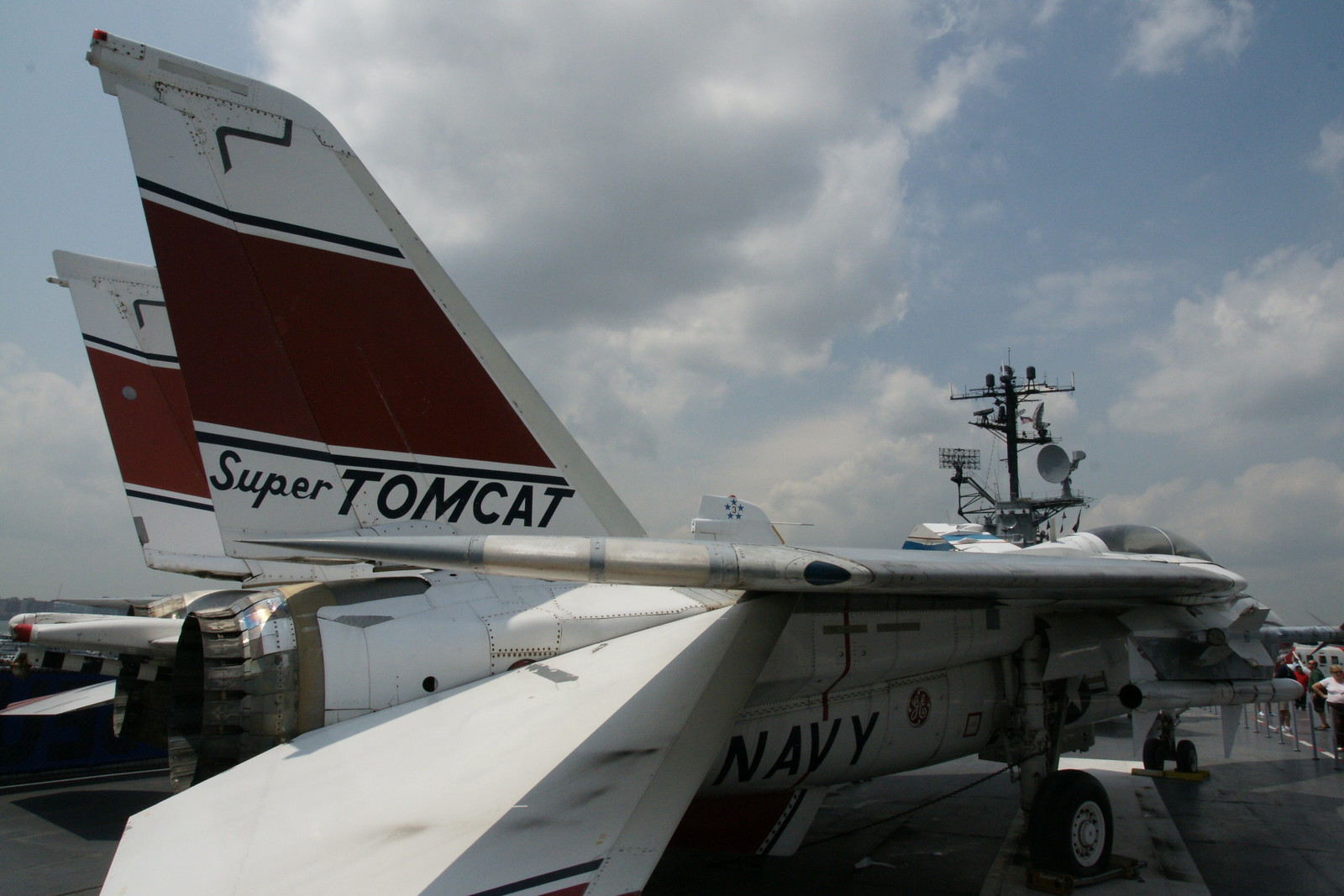The image features a Navy jet known as the "Super Tomcat," prominently displayed on what appears to be an aircraft carrier or military base under a blue sky filled with puffy clouds. The jet, mostly white and gray with large, extended wings, has a distinctive double tail on the left side. The tail features a central maroon stripe bordered by thin white stripes, topped with a darker, almost maroon section. The tail wing displays the words "Super Tom Cat" in black letters; "Super" is styled in cursive while "Tom Cat" is in bold block letters. On the right side near the bottom, the word "NAVY" is clearly visible in capital letters. The jet's front wheel, with a black tire and white center, is chocked for stability. The scene in the background includes possible radar sections and pylon antennas, suggesting a setting on an aircraft carrier.